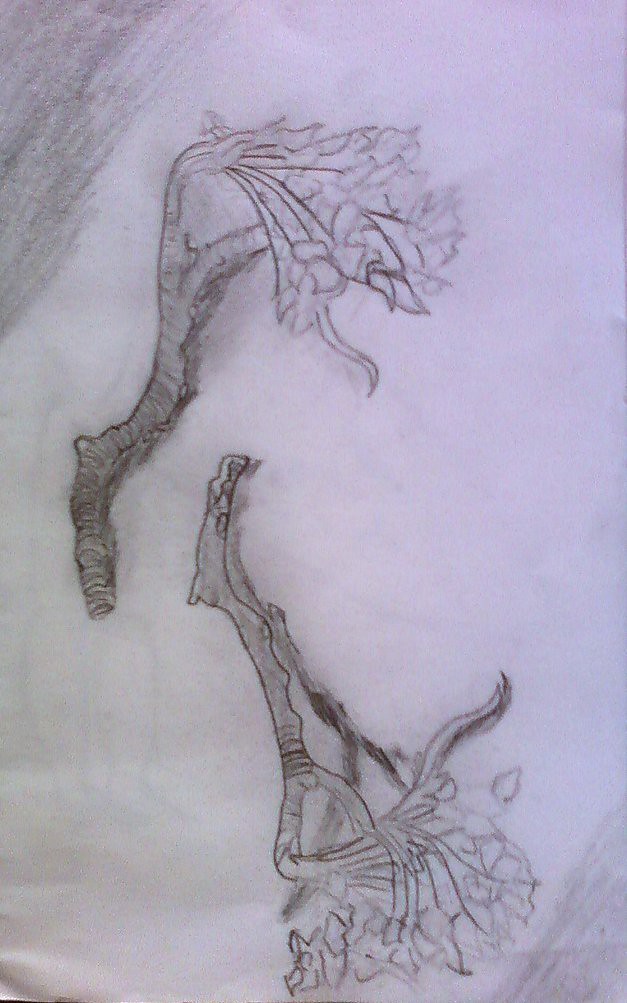This intricate pencil drawing beautifully portrays two delicate twigs or small branches adorned with numerous tiny flowers. The artwork is characterized by the careful attention to detail and the soft, organic lines that describe the natural elements.

Positioned diagonally, the composition features a prominent twig in the top left quadrant, stretching from the southwest to the northeast. This twig exhibits a gentle crook midway, where it goes up, bends slightly to the right, and then ascends further. Numerous secondary branches emanate from this main stem, each bearing small clusters of flowers, intricately sketched with subtle details to suggest their delicate petals. These blossoms, appearing to be about twelve to fifteen in number, add a sense of life and movement to the piece.

In parallel, a second twig emerges from the bottom right quadrant, extending from the northeast to the southwest. This branch, featuring a more pronounced crook to the right, also sends out smaller lateral branches. These extensions, adorned with loosely drawn leaves or flowers, extend horizontally and then gently droop downward, enhancing the sense of natural growth and gravity.

An additional, seemingly broken branch emerges from behind the flowers, extending back upwards in a northward direction. This element adds depth and complexity to the drawing, suggesting layers of growth and the resilience of nature.

The composition is framed by areas of pencil scribbling in the top left and bottom right corners, providing a contrasting background that highlights the detailed rendering of the twigs and flowers. The overall effect is a harmonious blend of structure and spontaneity, capturing the ephemeral beauty of blooming branches.